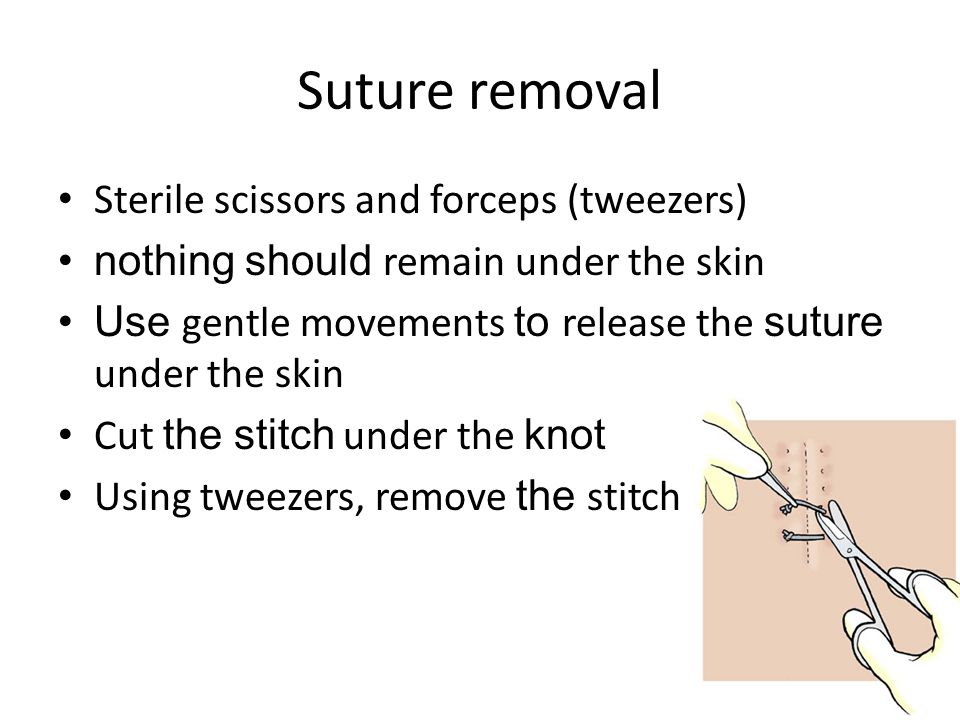The image is a slide from a PowerPoint presentation on suture removal, prominently featuring black text on a white background with a headline reading "Suture Removal." Below the headline, five bullet points provide detailed instructions: "Sterile scissors and forceps (tweezers)," "Nothing should remain under the skin," "Use gentle movements to release the suture under the skin," "Cut the stitch under the knot," and "Using tweezers, remove the stitch." In the bottom right corner, a color illustration shows two gloved hands performing suture removal, one holding tweezers to lift the stitch while the other uses surgical scissors to cut it. The image uses light colors, including black, white, yellow, and peach, to convey a clear, instructional approach, making it ideal for healthcare professionals.